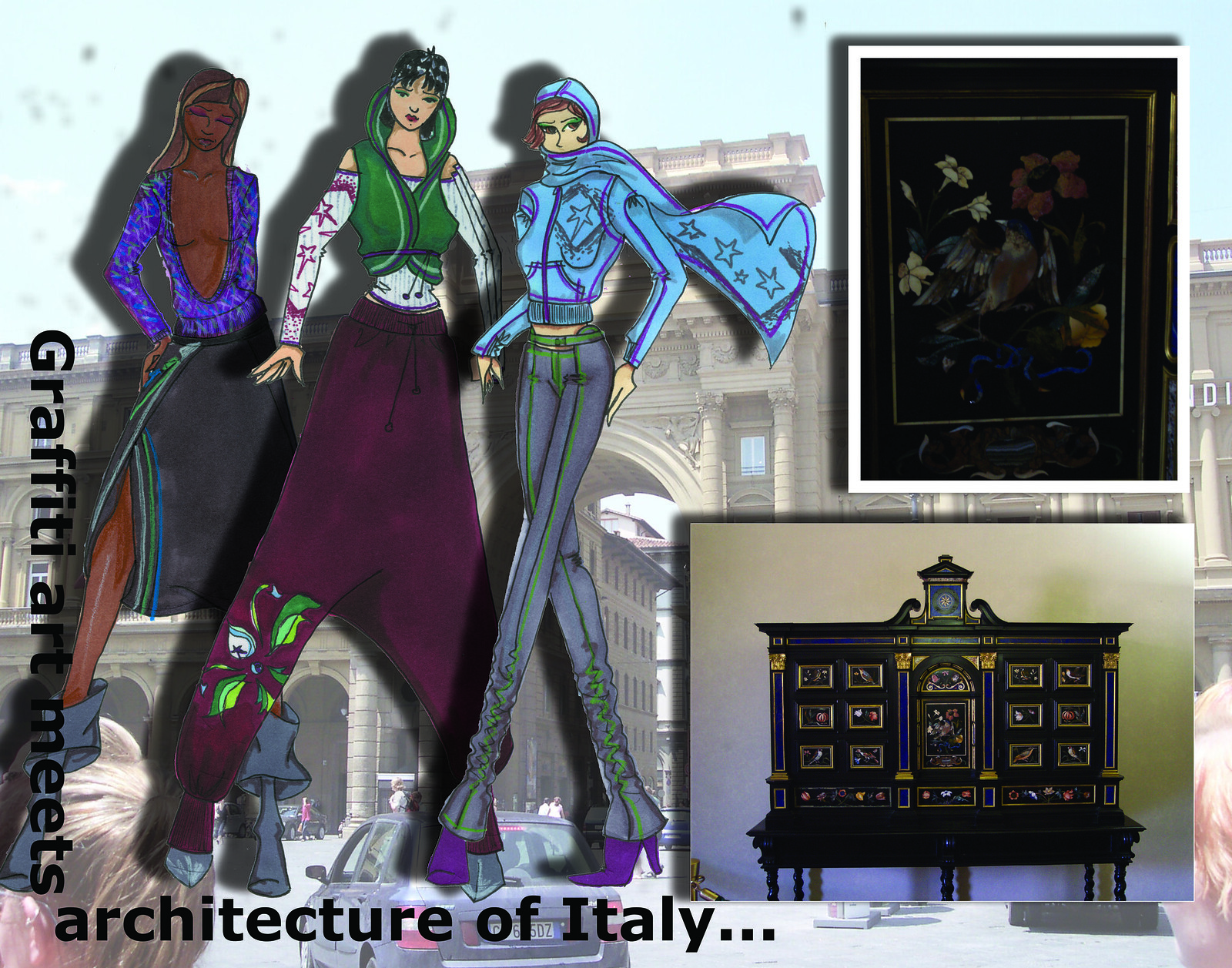The image is an intricate blend of anime-style artwork and real-life elements, creating a vivid scene labeled "graffiti art meets architecture of Italy." The left side features three tall, stylishly dressed women. The woman on the far left, a Black woman, dons a purple open-chest shirt paired with a black skirt detailed with green and blue lines, and blue boots. The middle woman, a White woman with black hair, wears a green vest over a white strapless shirt and purple pants. The woman on the far right, a red-haired White woman, sports a blue hooded jacket, a blue scarf adorned with stars, gray pants, and purple heels. The background showcases a busy Italian street adorned with monuments, buildings, and cars, adding a real-world touch to the animated subjects. On the far right, there is an elegant piece of furniture with multiple ornate drawers and a framed floral print with a dark matting and a gold-colored frame, adding to the picture's fusion of modern and classic artistic elements.